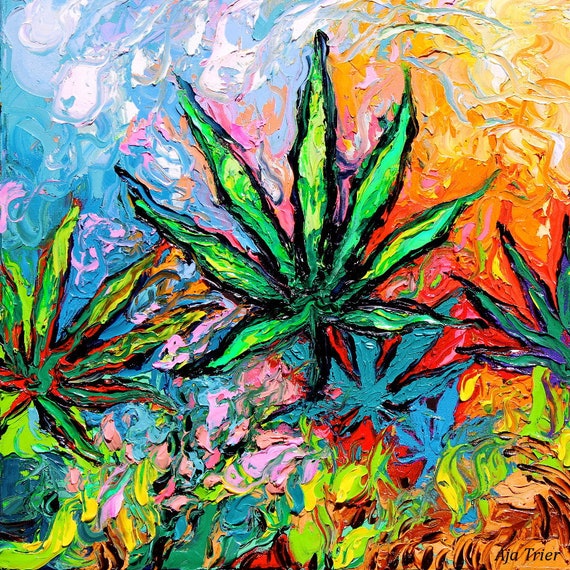This vivid oil painting features an abstract depiction of marijuana plants with a heavy emphasis on bright, swirling colors and thick, textured brush strokes. In the center of the composition, several marijuana leaves fan out with approximately seven long blades each, rendered in a variety of vibrant shades including greens, yellows, pinks, reds, blues, and teals. The background on the left side of the painting blends pink, blue, and white hues, evoking a sense of sky or water, while the upper right corner transitions into warm shades of red, orange, and yellow, reminiscent of a sunrise or sunset. The bottom part of the painting is a colorful medley, featuring an array of greens, yellows, pinks, reds, blues, browns, and oranges. The overall arrangement is abstract, with leaves scattered throughout and the colors swirling together in a 70s-inspired aesthetic. The artist's name is visible in the bottom corner, adding a personal signature to this dynamic and multicolored piece.